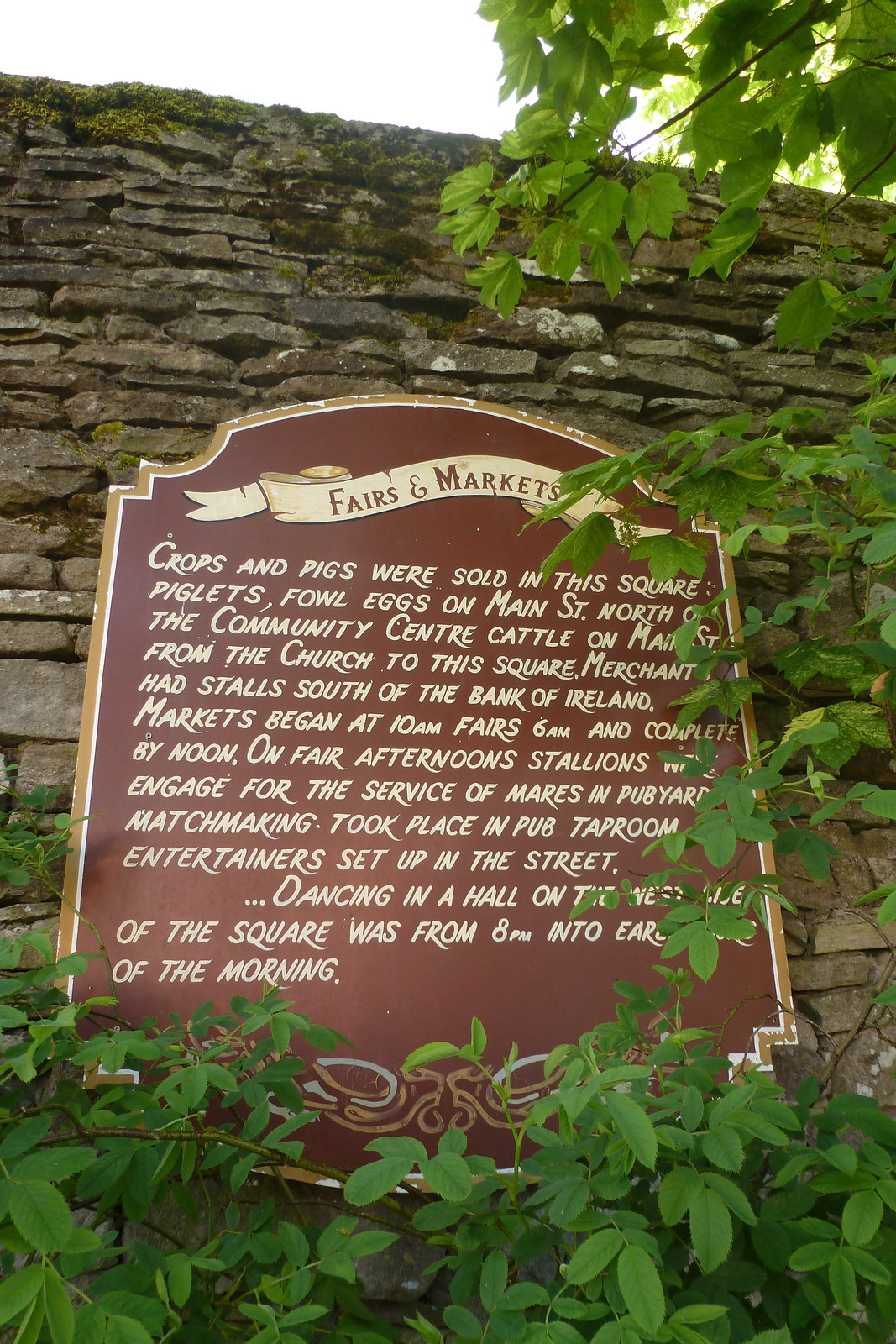The image depicts a historic commemorative plaque centered on a gray concrete wall, adorned with a red background, gold trim, and white text. This wall, composed of thin stone tiles, serves as the backdrop for the plaque. Surrounding the plaque are green plants and leaves, with bushes positioned below and some overhanging foliage on the right. The plaque details the vibrant activities of past fairs and markets: crops and pigs in the square, piglets and fowl eggs on Main Street north of the community center, cattle from the church to the square, and merchants' stalls south of the Bank of Ireland. It notes that markets began at 10 a.m., while fairs started at 6 a.m. and concluded by noon. Fair afternoons featured stallions engaging for the service of mares, public yard matchmaking in the pub taproom, entertainment set up in the street, and dancing in the hall from 8 p.m. into the early morning. This image captures a slice of history, vividly illustrating the lively commerce and community interactions of a bygone era.